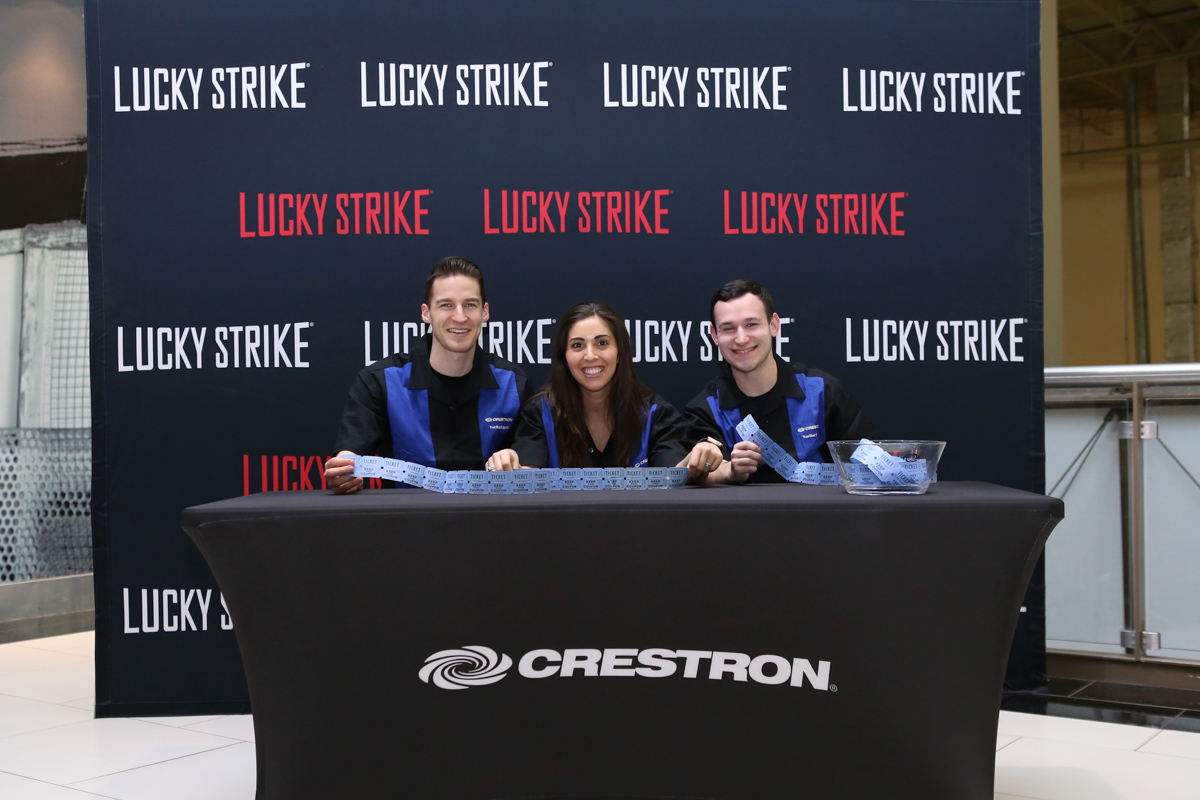In the photograph, a set resembling a TV show or sales convention booth is depicted. Three individuals, sporting matching blue vests over black shirts, are seated at a cloth-covered desk that bears the white Crestron logo and text. Positioned between them on the gray table is a bowl filled with tickets, which they are actively holding in their hands, suggesting a raffle or lottery event. The setup appears designed for video recording, as evidenced by the backdrop which prominently features the "Lucky Strike" logo repeatedly in alternating rows of white and red font over a dark backdrop. The background further reveals a partitioned area with metal railings and a glimpse of walls, bricks, and pipes beyond the partitions. The trio consists of two men with brown hair flanking a woman, also with brown hair, who sits in the center. They are all smiling, possibly engaging on behalf of Crestron at what could be a promotional or competitive event.